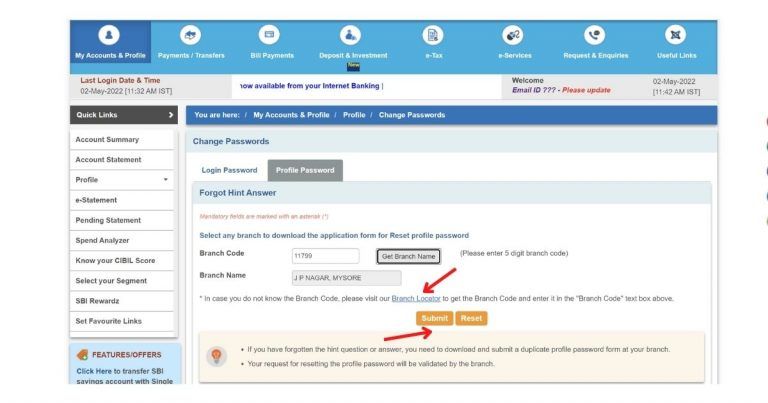The image captures a detailed screenshot of an internet banking website. The top section prominently displays navigational options including "My Account and Profile," "Payments and Transfers," "Bill Payments," "Deposit," "E-Tax," "E-Services," "Requests," and "Useful Links." Notably, it indicates the user's last login date as May 2nd, 2022, emphasizing its status as a portal for online banking.

A welcoming message prompts the user to input their email ID and highlights the necessity to update certain information, marked in orange. A quick links section is situated below, providing shortcuts to various features such as "Account Summary," "Account Statement," "Profile Statement," "Pending Statement," "Spend Analyzer," "Know Your CIBL Score," "Select Your Segment," "SBI Rewards," and an option to "Set Favorite Links."

The website offers special features, also highlighted in orange. The user's current location within the site is indicated as "My Accounts and Profile," specifically under "Profile and Change Passwords." A blue bar beneath it outlines options to change passwords, dividing them into "Login Password" and "Profile Password," with the latter grayed out for differentiation. 

A light blue bar features the option to "Forgot Hint Answer," while another orange annotation, though too small to decipher, occupies the center. It includes an option to select any branch for downloading the application form necessary to reset the profile, pointing out the requirement for a branch code and name with the instruction to "get branch here" clearly emphasized in bold black text accompanied by an arrow.

The process for entering a five-digit branch code is marked with a red arrow leading to the "Branch Locator," highlighted in blue. Below this, there are buttons for "Submit" and "Reset," illustrating the procedure for users who have forgotten their hint question or answer. It instructs them to download and submit duplicate profile password forms at their respective branches. The final note details that any request related to the profile password will need to be validated by the branch.